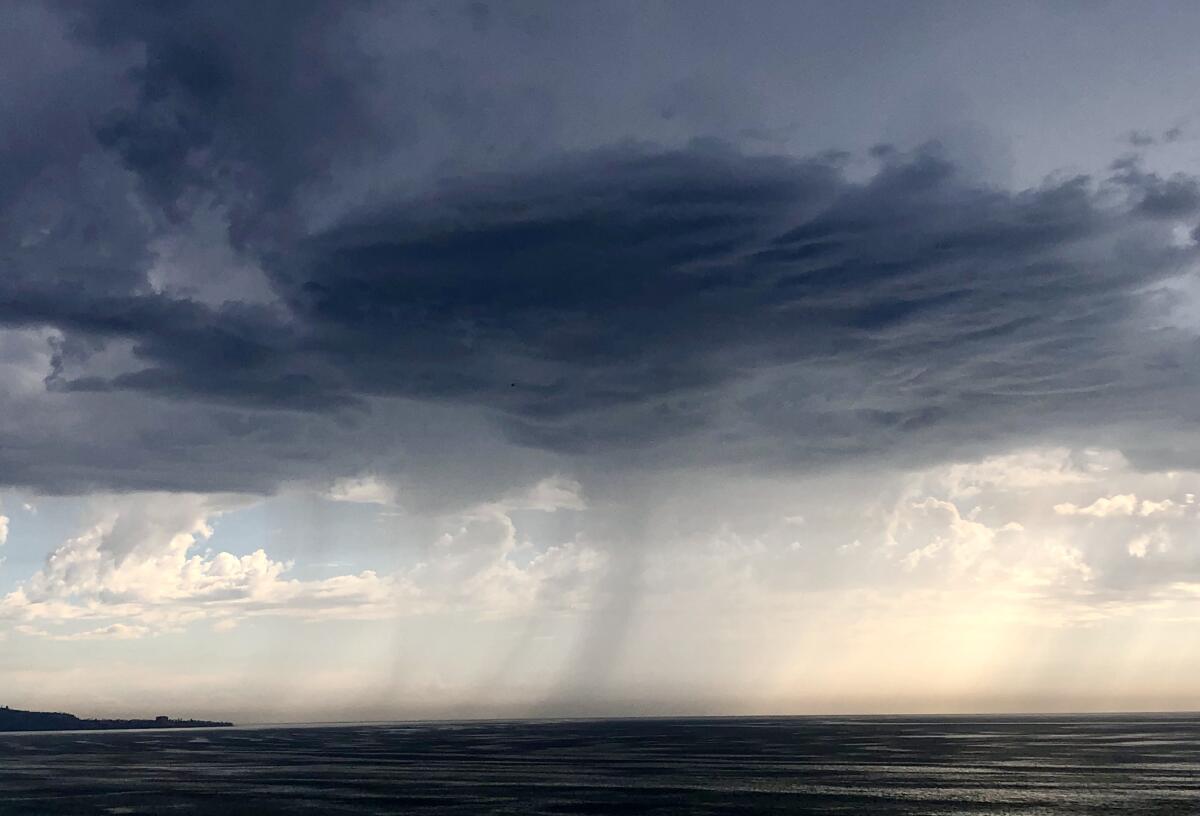The photograph captures an outdoor scene dominated by a stormy sky over a water expanse, which could be the ocean or a large lake. The image is wider than it is tall, with the water taking up a thin strip at the bottom. This water area appears dark gray or dark blue, possibly indicating turbulent conditions. On the left side, a small, indistinct peninsula or island extends outward, occupying about one-fifth of the frame.

The sky above the horizon begins with a lighter section where sunlight can faintly be seen filtering through fluffy white clouds. This gives way to a dramatic expanse of dark, ominous storm clouds, which occupy the top half of the image. The storm clouds are particularly dark and dense in the middle section.

Vertical streaks of gray, suggestive of heavy rainfall, descend from these clouds and curve slightly to the left, resembling tornado-like shapes but without forming actual funnels. This curvature implies the influence of strong winds. Overall, the image conveys a powerful sense of nature's intensity, with a stark contrast between the lighter lower sky and the foreboding storm above.